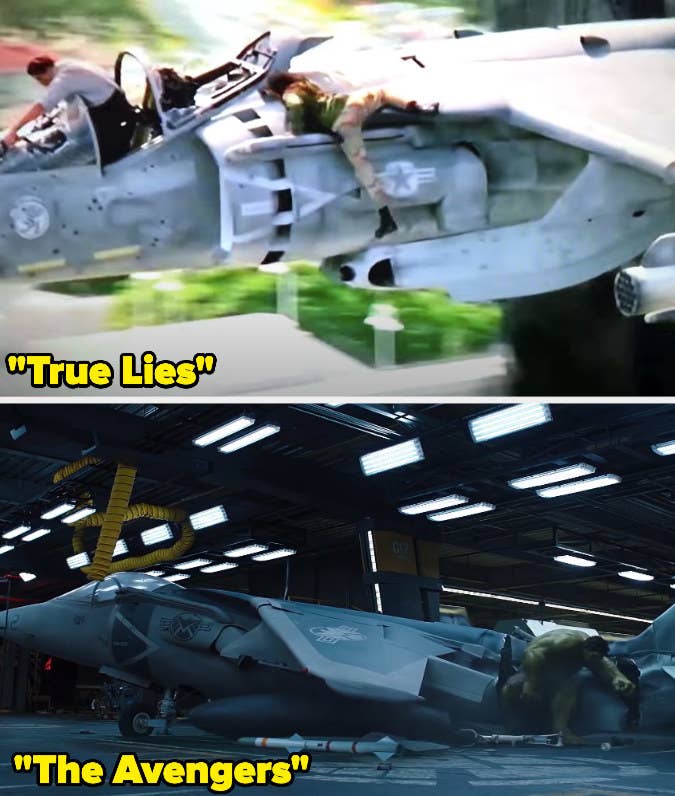The composite image consists of two horizontal frames stacked vertically, each depicting a scene from different action movies, captured in high detail. The top frame is from the movie "True Lies," with the title appearing in yellow text with quotation marks in the bottom left corner. This frame captures a tense moment with a jet in mid-flight. A pilot in a white shirt and dark pants is stationed in the cockpit, while another figure, possibly a soldier or operative in light green attire, perilously climbs over the aircraft's nose. The background is blurred to emphasize motion and danger. The second frame, labeled "The Avengers" in matching yellow text with quotation marks, illustrates a more chaotic scene. Here, the Hulk, recognizable by his green hue, is seen emerging from a damaged jet inside what looks like a dimly lit hangar. The hangar features a cement floor, fluorescent lighting, and a conspicuous yellow spiral tube in the upper left corner. Both frames are well-spaced, emphasizing the dramatic action and high-stakes scenarios common in both films. Each scene is rich in contrasting colors, including shades of gray, green, yellow, black, orange, white, red, and pink, enhancing the visual impact.